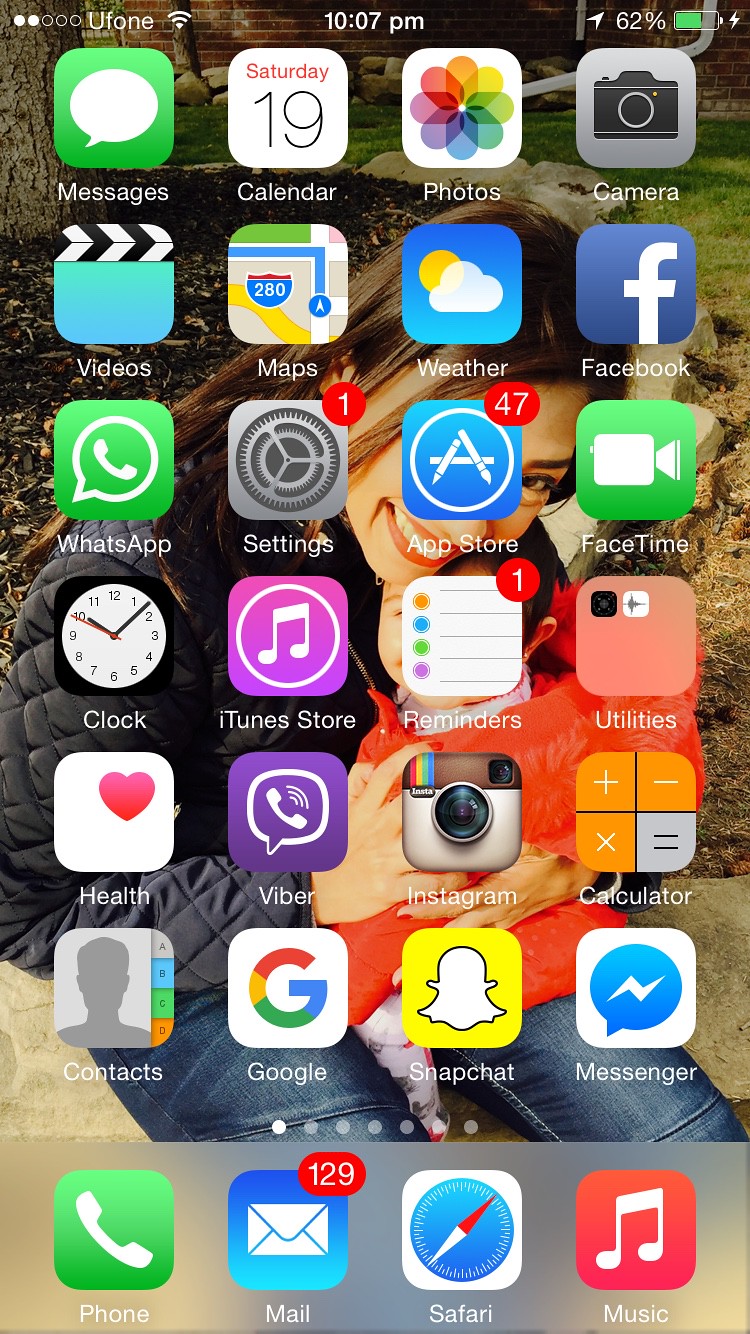This image is a detailed screenshot of the apps displayed on a mobile phone’s home screen. The background wallpaper features a woman with long, straight brown hair holding a baby tenderly in her arms. She is smiling, wearing lipstick, and dressed in blue jeans and a puffy, quilted black jacket. She is seated, with her thighs partially visible at the bottom of the picture. The setting appears to be a garden, visible in the background with bark at the base of a tree on the left, decorative rocks encircling the tree, and a brick house behind with additional decorative rocks in the front. There is also grass visible to the right.

The app icons are organized into six rows, each containing four apps, with several notifications visible. The first row features the 'Messages' app. Following this are 'Calendar,' 'Photos,' 'Camera,' 'Videos,' 'Maps,' 'Weather,' 'Facebook,' 'WhatsApp,' and 'Settings' – the 'Settings' app has a single notification marked by a white number on a red background. Next is the 'App Store,' which shows 47 pending notifications. The fourth row has 'FaceTime,' 'Clock,' 'iTunes Store' with one notification, and 'Utilities.' The fifth row includes 'Health,' 'Viber,' 'Instagram,' and 'Calculator.' The sixth row contains 'Contacts,' 'Google,' 'Snapchat,' and 'Messenger.' At the bottom of the screen are the essential apps: 'Phone' icon, 'Mail' icon with 129 unread messages, 'Safari' icon, and 'Music' icon.

This vivid description captures the image's intricate details, both of the background and the arrangement of the apps on the mobile device.